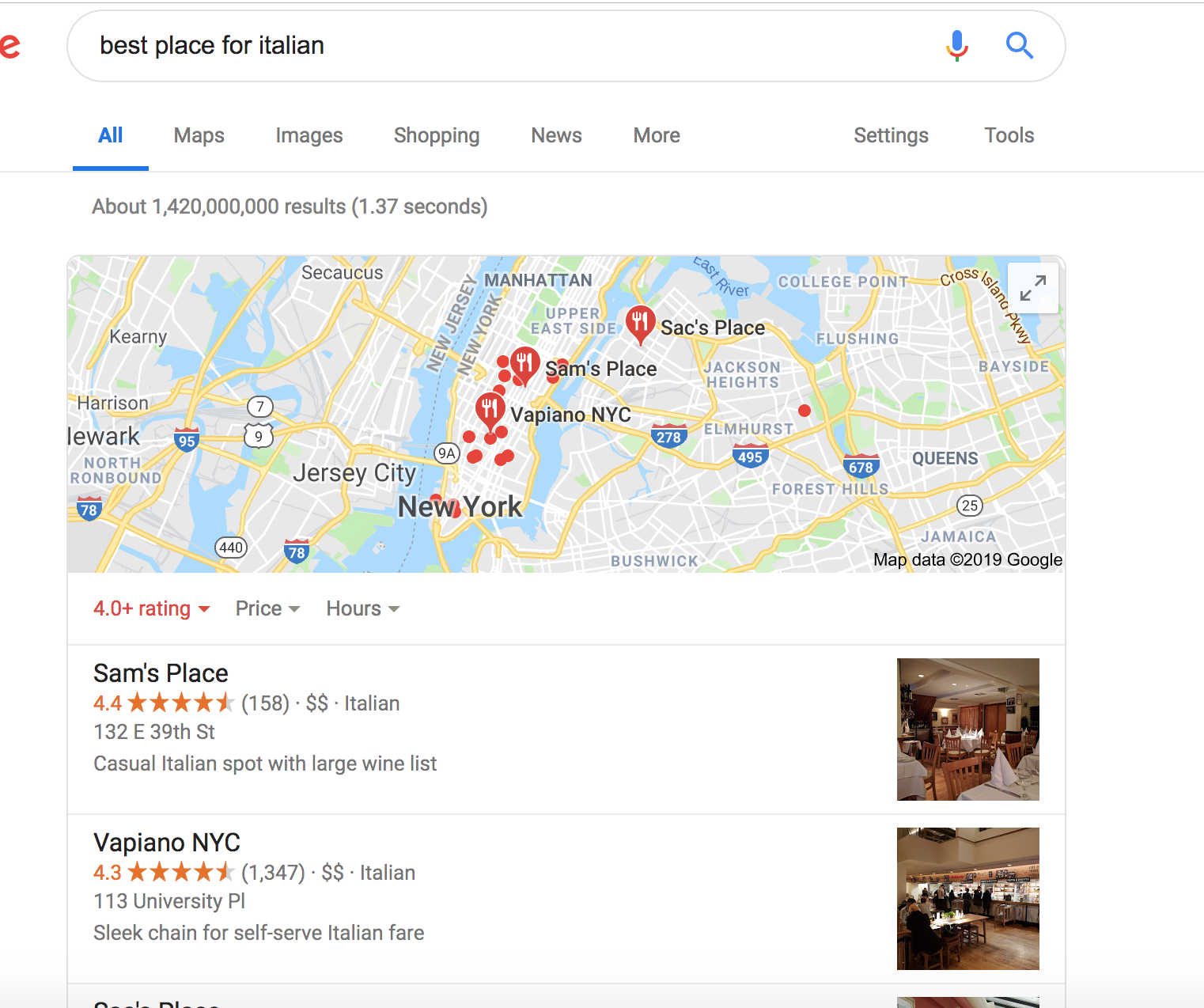The image depicts a webpage from a search engine, focused on finding the best places for Italian cuisine. At the top of the page, there is a search bar displaying the query "best place for Italian," accompanied by a microphone icon for voice search.

The main navigation option highlighted is "All," marked in blue (A-L-L) with a blue underline, indicating it is the selected filter. Below this, there is a map with red pins, each featuring a fork and knife symbol, representing various Italian restaurant locations in New York City, including areas like Queens and Brooklyn.

Two specific restaurants are featured prominently:

1. **Sam's Place**:
   - **Rating**: 4.4 out of 5 stars, indicated by a label in red displaying a "4.0+ rating" with a dropdown for more filters.
   - **Description**: Casual Italian spot with a large wine list.
   - **Visual**: Includes a photograph of the restaurant's elegant setting, complete with tablecloths and cloth napkins.

2. **Vapiano, New York City**:
   - **Description**: Sleek chain known for self-serve Italian fare, resembling a buffet-style service.
   - **Visual**: A photograph depicting the self-serve setup.

Both establishments are presented within white information boxes. Additionally, there are grey tabs for filtering results by "Price" and "Hours."